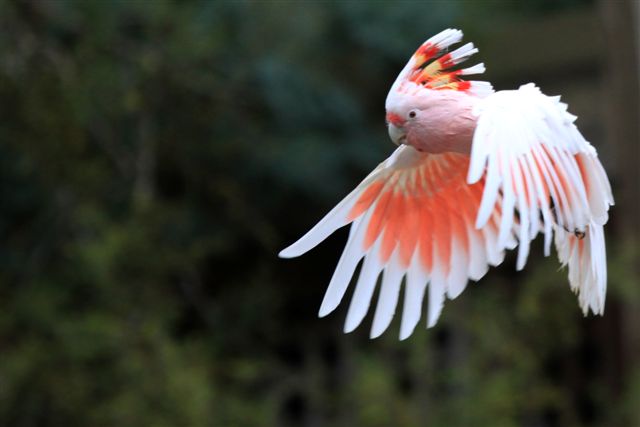The image shows a strikingly colorful bird in mid-flight, positioned towards the upper right corner of the frame and facing left. The bird's wings are outstretched, with the right wing’s inner feathers displaying a gradient from white to a soft peach, and hints of red and orange toward the tips, while the outer side of the left wing remains predominantly white. The bird's body and tail feathers are mainly white, but the tail also shows some red. Its head is quite vibrant, featuring a combination of colors: the base of its head feathers is yellow, transitioning to red, with the very tips being white. The face is light pinkish with a distinctive red band just above its white beak. The bird's eye is sharp with a black pupil and a white iris. The background, although blurred, clearly depicts a dense setting of trees, twigs, branches, and varying greenery, allowing the vividly detailed bird to stand out prominently in the foreground. The overall composition suggests either a highly detailed photograph or a computer-generated image emulating photographic realism.